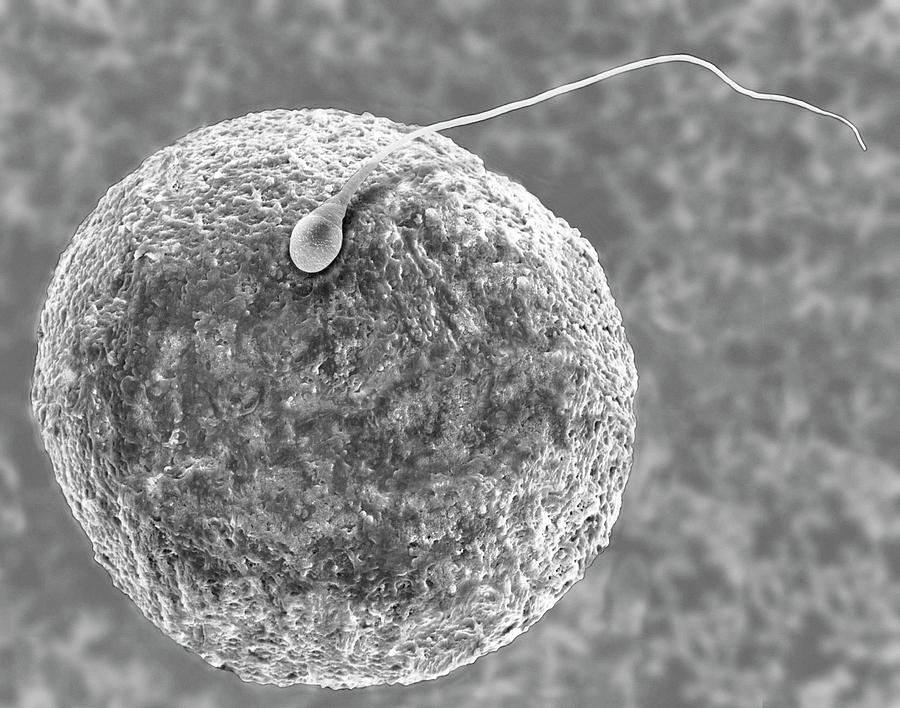This highly detailed black and white microscopic image captures a pivotal moment of fertilization, depicting a sperm cell poised to penetrate a human egg. The large textured ovum, resembling a roughly spherical globe with bumpy indentations, occupies approximately 60-75% of the image, dominating the left side. The texture of the egg resembles that of a sponge or cantaloupe skin, with the central area of the egg appearing darker gray and the outer edges lighter. Resting towards the top center of the egg, the sperm cell is distinctly visible, its head in direct contact with the egg surface. The sperm's long tail extends upward to the right, with some descriptions noting a slight curvature toward the end. The background of the image is blurred with a similar gray and white coloration and texture, enhancing the focus on the detailed interaction between the sperm and the egg. The overall high-resolution quality of the image reveals the sperm cell either preparing to penetrate or just establishing initial contact with the egg, highlighting the initial steps of conception.